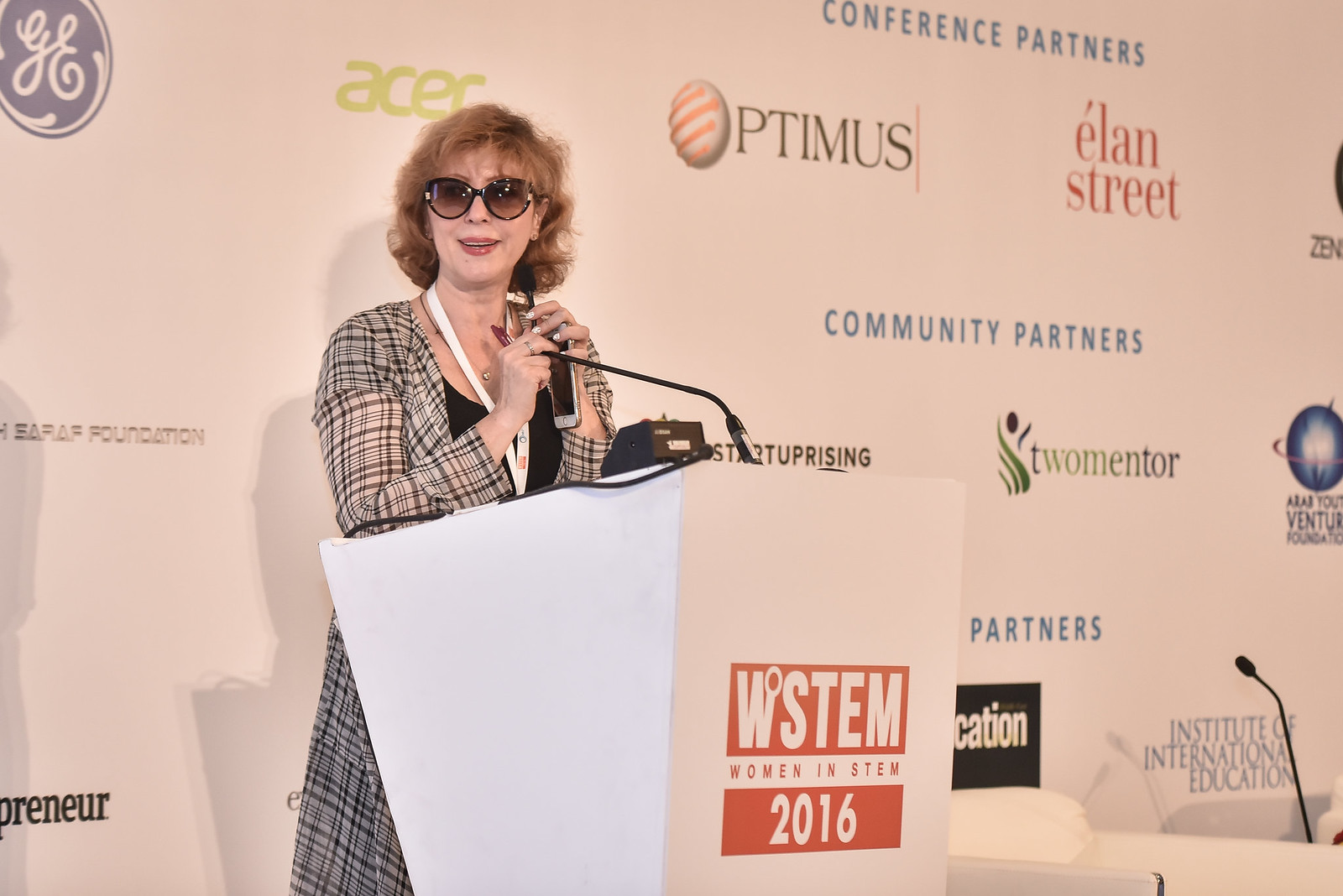The image captures a light-skinned woman with short brown hair, wearing rose sunglasses and a checkered brown and white jacket over a black top, standing at a podium. She is speaking or perhaps answering questions at a STEM conference, and she has her hands around a wired microphone in front of her. Around her neck, she has a lanyard with identification. Behind her is a large white backdrop scattered with various company names, such as GE, ACER, Elan Street, and Community Partners. Noticeably, "Conference Partners" is repeated in blue, while the word "Optimus" with a distinctive egg-shaped 'O' featuring horizontal red lines is prominently displayed. The podium she stands behind is white, with two red rectangles on the front, one stating "WSTEM" and another below it indicating "2016" in thin white lettering. The phrase "Women in STEM" is subtly written against the white background between the two red rectangles. The scene is professional and imbued with a sense of engagement and positivity, as she smiles and looks slightly to the left.